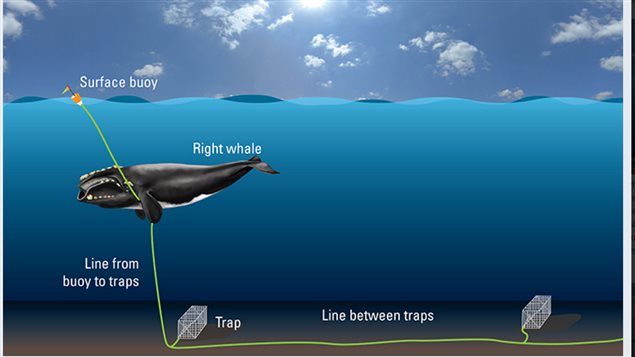The rectangular image, measuring approximately 4 to 5 inches wide by 3 inches high, showcases an underwater scene framed by a thin vertical black line and a slightly thicker inner gray line on the right side. The scene begins at the lower half-inch of the image, displaying a brown seafloor bed topped by dark blue water. Ascending from the seafloor, the water transitions from a dark blue to a medium blue midway up the image, culminating in a sky filled with scattered white clouds and a radiant, white sun at the top center.

On the surface of the water, in the upper left section, an orange buoy with an orange flag is labeled "Surface Buoy" in white text. This buoy is attached to a green line leading to a right whale in the water below. The whale, depicted as gray with a white underbelly and markings around its face, seems entangled in the line, which is clearly labeled in the image as "line from buoy traps." The green line extends down to the seafloor, where it connects two traps lying on the sand. Each trap is indicated with the label "line between the traps." The entire composition, enhanced by the detailed labeling and visual elements, vividly portrays the entanglement of the whale and the placement of the traps on the ocean floor.